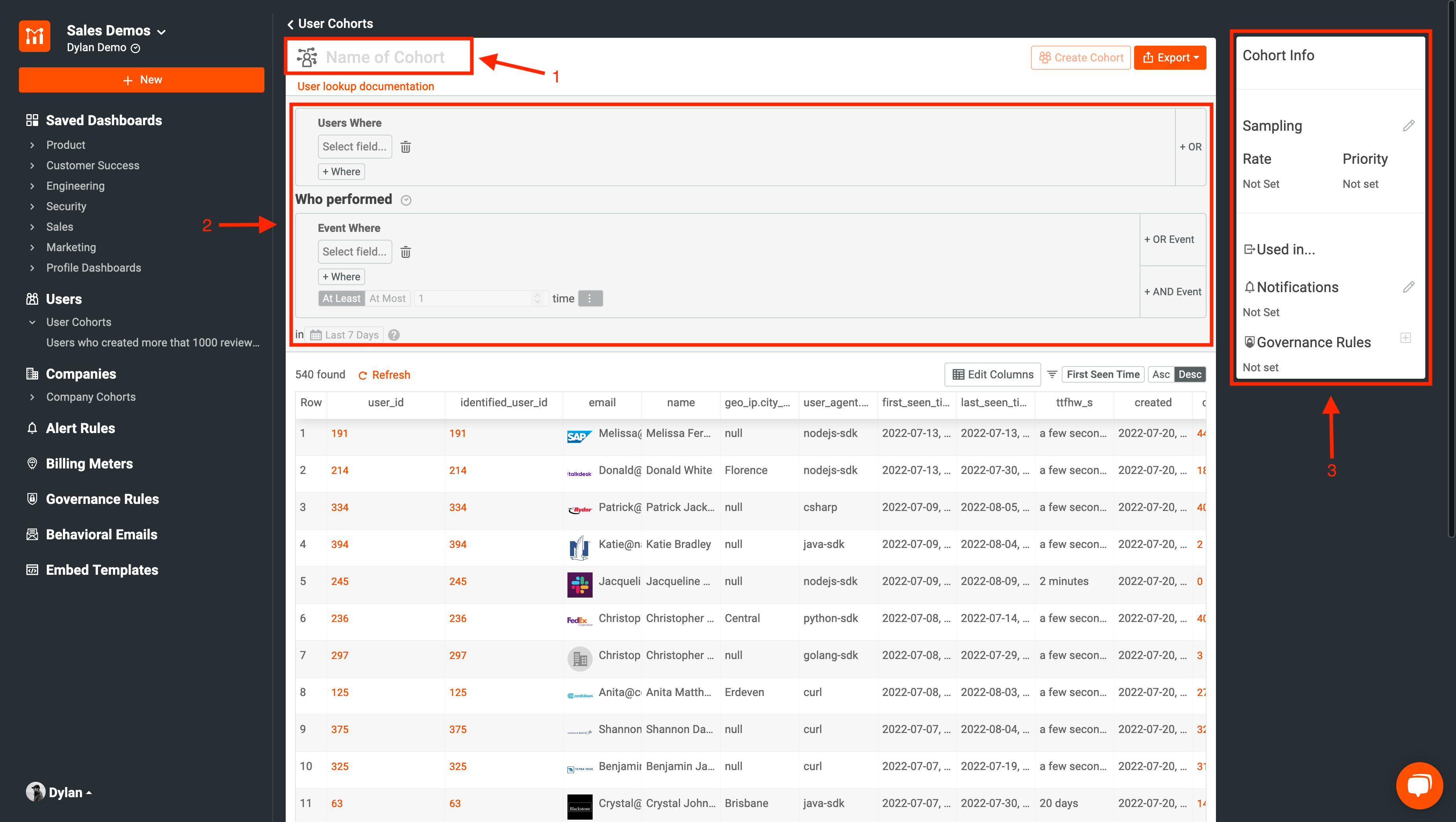The image features a detailed user interface layout. In the top-left corner, there is a small black box. Adjacent to it, to the right, is an orange square featuring a design that resembles the letter "M" and the text "Cell Demo, Dillon Demo." Below this section, an orange rectangle labeled "New" is prominent. Following this are a series of labels listed one after the other: "Save Dashboards," "Product," "Customer Success," "Engineering," "Security," "Sales," "Marketing," and "Profile Dashboards." 

Beneath this, additional categories are listed: "Users," "User Cohorts," "Users who created more than 1,000 reviews," "Companies," "Company Cohorts," "Alert Rules," "Billing Meters," "Governance Rules," "Behavior Emails," and "Embed Templates."

On the right side of the image, there is a section marked with the heading "Name a Cohort," and a notable red arrow is pointing at this title. Just below, there is a note stating "User Lookup Documentation." Further down, the text "Users Where" can be seen above a box labeled "Select Field," accompanied by a trash icon. Below this box, it appears to be leading into another section that begins with the word "Where."